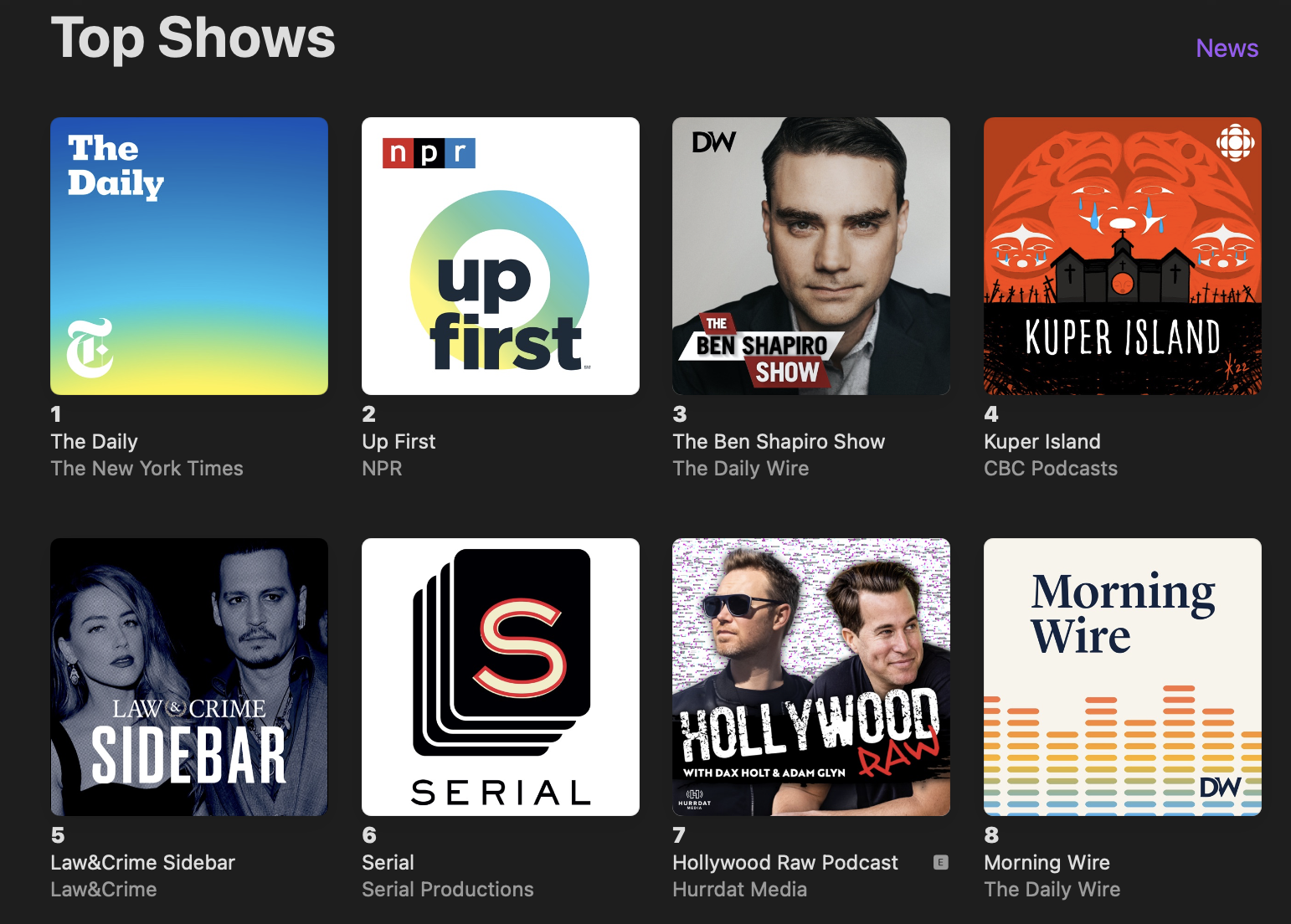The image features a black background displaying various podcast logos organized in two rows of four. 

- In the top left corner, bold gray text spells out "Shows" with a capital "S".
- On the right side, in smaller purple text, it says "News".

### Top Row:
1. **First Logo:**
   - A blue square with a strip of yellow at the bottom.
   - "The Daily" is written in the top left corner, with the New York Times emblem in the bottom left.

2. **Second Logo:**
   - A gray square.
   - "The Daily" and "The New York Times" are written in sequence.

3. **Third Logo:**
   - A white square featuring smaller red, black, and blue squares in the top left.
   - "NPR" is written in the top left corner.
   - A blue circle that transitions to yellow on the left side.
   - "Up First" is written in big black letters at the center, with a smaller "Up First" and "NPR" underneath.

4. **Fourth Logo:**
   - The Ben Shapiro Show.

### Bottom Row:
1. **First Logo:**
   - Law & Crime.
   - "Sidebar" is written in big bold text beneath it.

2. **Second Logo:**
   - Serial.

3. **Third Logo:**
   - Hollywood Raw with Dax Holt and Adam Glyn.

4. **Fourth Logo:**
   - Morning Wire.